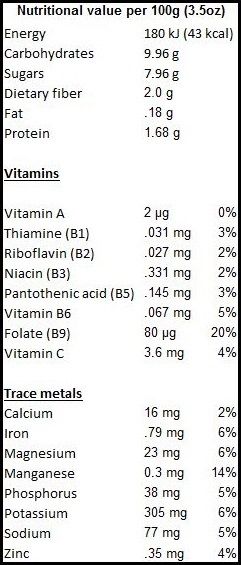This image displays a meticulously cropped, rectangular nutritional label without any extraneous details, suggesting it's a screenshot from an online source. The label features a thin black border and is set against a white background. The text is predominantly in black, with certain sections bolded for emphasis. At the top, it specifies the nutritional value per 100 grams (3.5 ounces), listing energy, carbohydrates, sugars, dietary fiber, fat, and protein. The label is organized into two main sections: the first includes vitamins such as Vitamin A, Thiamine (B1), Riboflavin (B2), Niacin (B3), Pantothenic Acid (B5), Vitamin B6, Folate (B9), and Vitamin C. The second section, outlined under "Trace Metals," lists calcium, iron, magnesium, manganese, phosphorus, potassium, sodium, and zinc. This detailed nutritional information suggests the label is from a food product or vitamin supplement, typically found in the pharmacy section of a store.